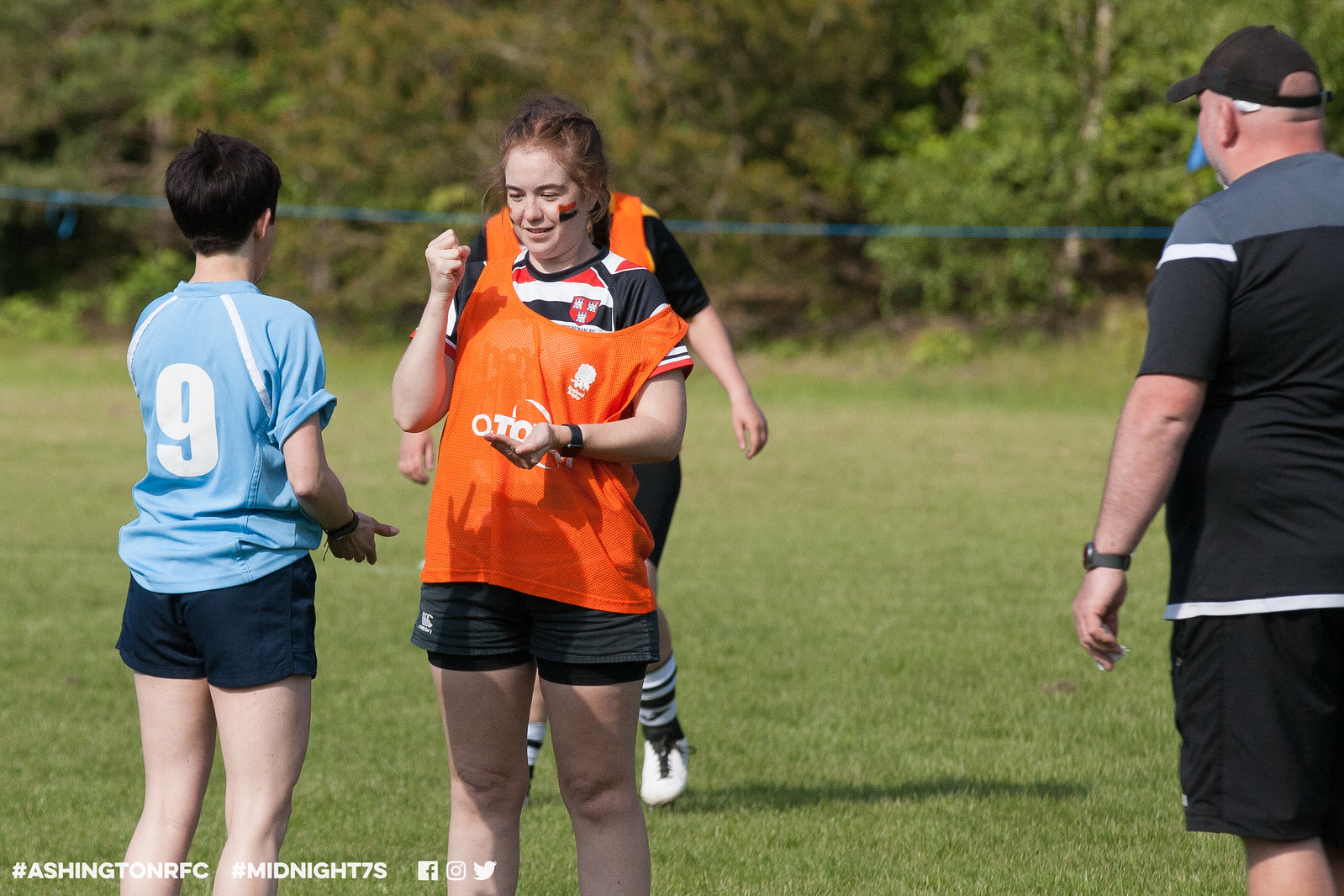The photograph captures a moment from a girls' soccer game where two players are engaged in a game of rock-paper-scissors, likely to determine who will start with the ball. On the left, a white girl with short black hair, styled almost like a boy's haircut, wears a light blue shirt with the number nine on it and black shorts. Facing her is another white girl with reddish-brown hair tied back in a braid, dressed in an orange pinnie over a red, white, and black shirt, and black shorts. To the far right of the frame, a man in a black baseball hat, black and gray shirt, black shorts, and a watch, presumably the coach, observes the scene. The backdrop consists of a green field, and in the bottom left corner, hashtags #AshingtonRFC and #Midnight7S are visible, alongside Facebook, Instagram, and Twitter logos.